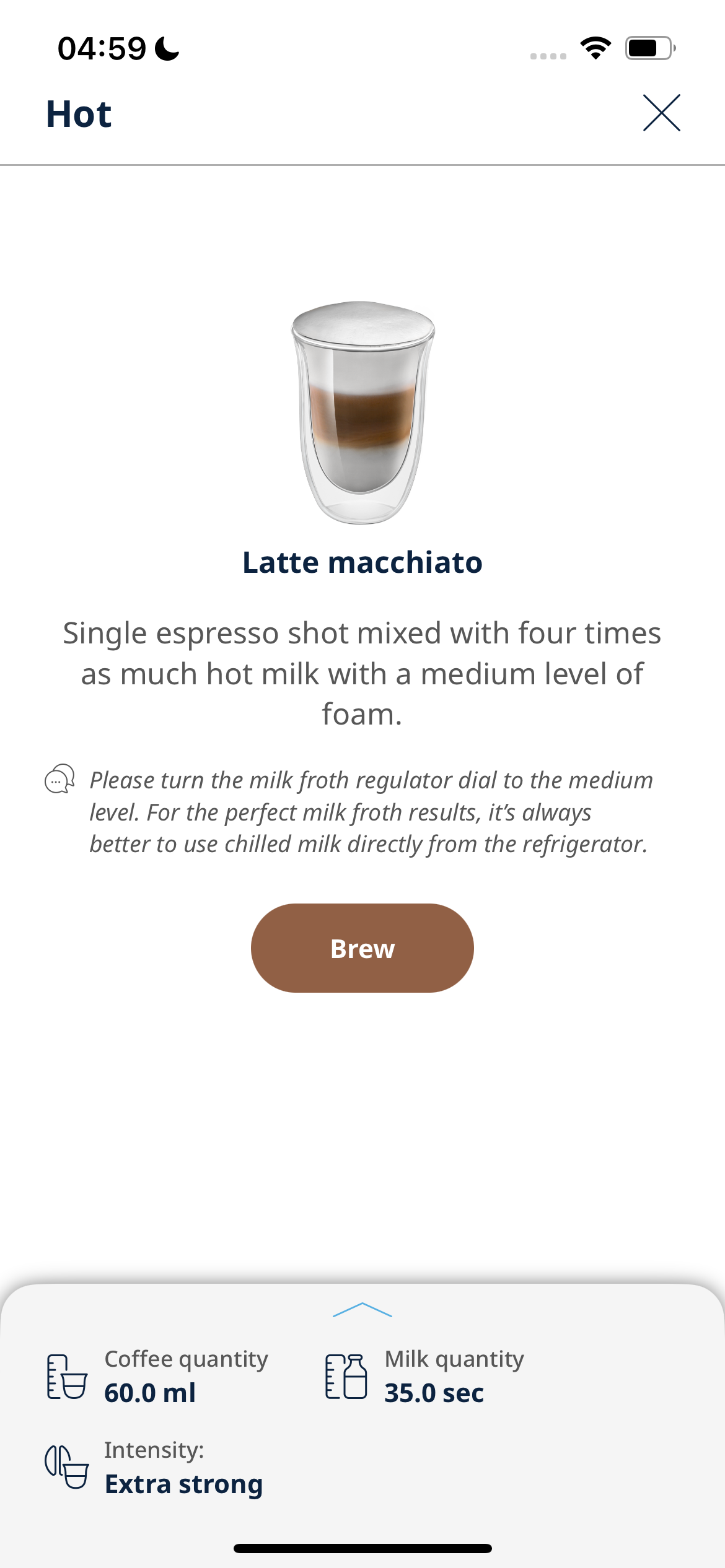This is a detailed screenshot of a cell phone display at 4:59 AM, identified by the small moon icon next to the time. The top right corner of the screen shows a full Wi-Fi signal and a battery indicator at approximately 75% charge. Below this, there is a status bar labeled "hot" and an X button to close the current screen.

The main part of the display features an image of a latte macchiato with the text "Latte Macchiato" below it. Further down, there is a description: "Single espresso shot mixed with four times as much hot milk with a medium level of foam." 

Following the description, there are instructions that read: "Please turn the milk froth regulator dial to the medium level for the perfect milk froth results. It's always better to use chilled milk directly from the refrigerator."

At the bottom of the screen, there is a brown 'Brew' button in white letters. Below this button, there are details that resemble a recipe or brewing settings: "Coffee quantity: 60 milliliters, Milk quantity: 35 seconds, Intensity: Extra strong."